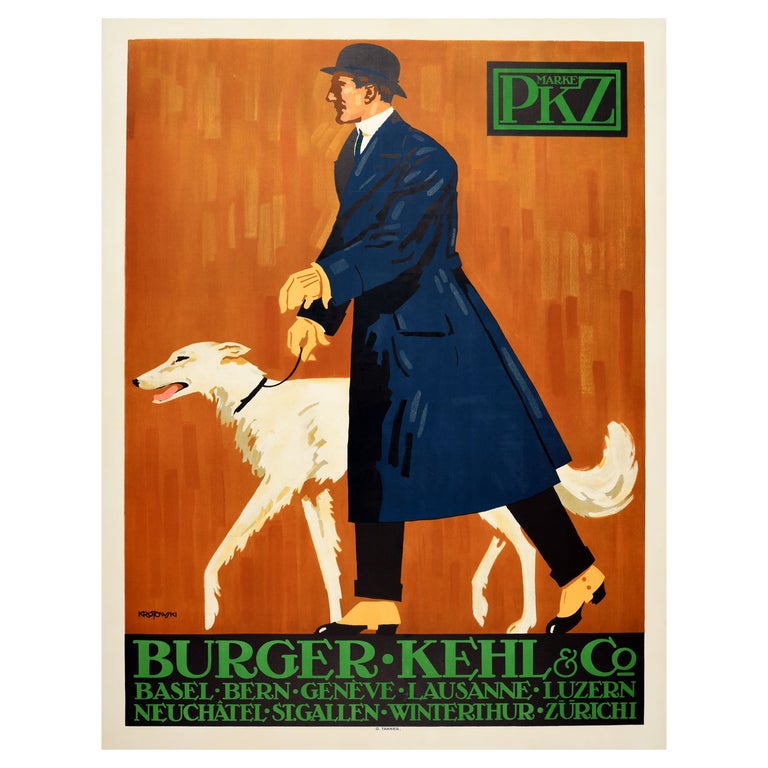This vintage poster, likely from the 1950s or early 1960s, exudes an air of sophisticated elegance. Dominated by an orange background, the poster features an animated man in a blue coat, blue tie, blue hat, black pants, and yellow formal shoes. The man is also wearing brown gloves and is walking towards the left with a slender, fully white dog by his side. The upper-right corner showcases a logo that reads "Marke PKZ" and beneath this, text appears listing "Berger, Kell and Company" followed by a series of Swiss cities including Basel, Bern, Geneve, Lausanne, Luzerne, Neuchatel, St. Gallen, Winterthur, and Zurich. The overall design and style suggest a high-class advertisement, evocative of classic movie or play posters from the mid-20th century.